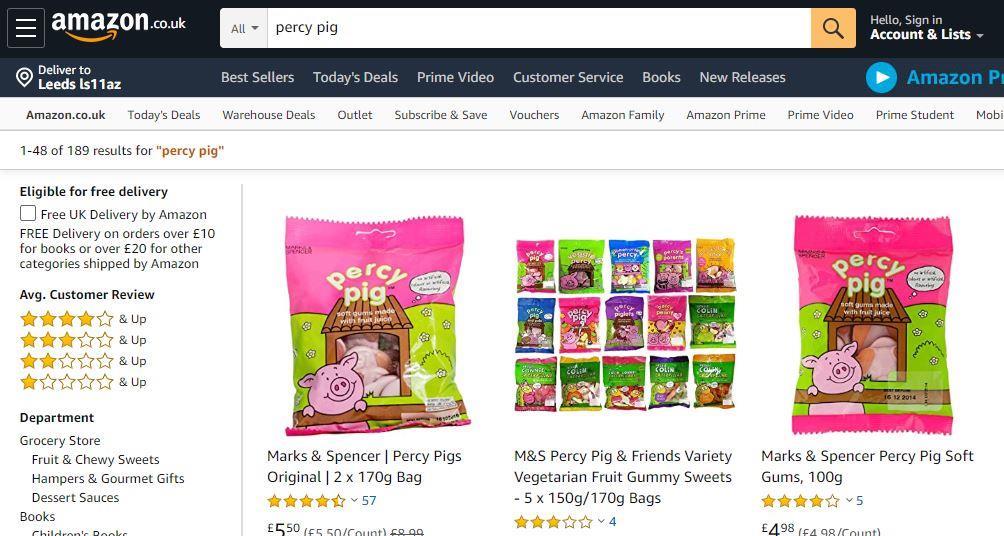This is a descriptive caption for an image of an Amazon search results page, showcasing products available for users in the UK:

---

This screenshot displays an Amazon.co.uk search results page for "Percy Pig." In the top right corner, the website URL confirms it's the UK version of Amazon. The search term "Percy Pig" has been entered into the search bar, revealing three main product listings:

1. **Marks and Spencer Percy Pigs Original**: This product consists of two 170-gram bags and has received a rating of 4.5 stars from 57 reviews. It is priced at $5.50.
2. **M&S Percy Pig and Friends Variety Vegetarian Fruit Gummy Sweets**: This option has a 3-star rating based on four reviews, but there is no visible price listed.
3. **Marks and Spencer Percy Pig Soft Gums (100 grams)**: This item is rated 4 stars from five reviews and is available for $4.98.

The page highlights that the user is viewing items 1 through 48 out of 189 total results for "Percy Pig," with many options eligible for free UK delivery. Details about free delivery include eligibility for orders over $10 for books and over $20 for other categories, shipped by Amazon. The page also allows users to filter results based on customer reviews, with options to see products rated with four stars and up, three stars and up, two stars and up, or one star and up.